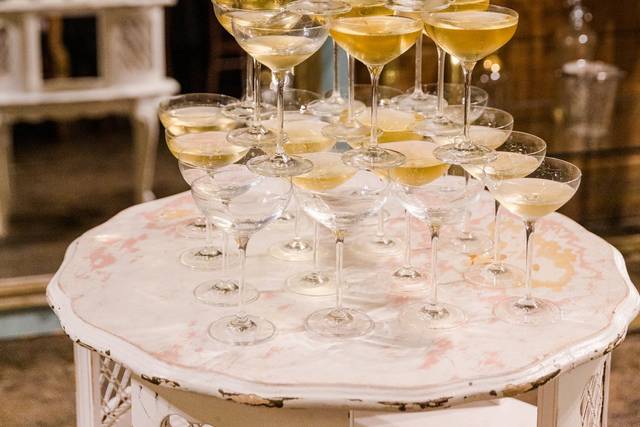The image captures a meticulously arranged champagne tower on a vintage, slightly distressed circular table. The table, cream-colored with hints of pink and light orange designs, features grooved edges and worn brown spots, suggesting an antique look. Multiple tiers of champagne glasses, some filled with a golden liquid, stand balanced atop each other. The glasses, characterized by their wide rims and shorter stature, form a cascading pyramid. The background appears out of focus, hinting at additional tables but drawing attention to the central champagne display, suggesting it was purposefully set up for this photograph.